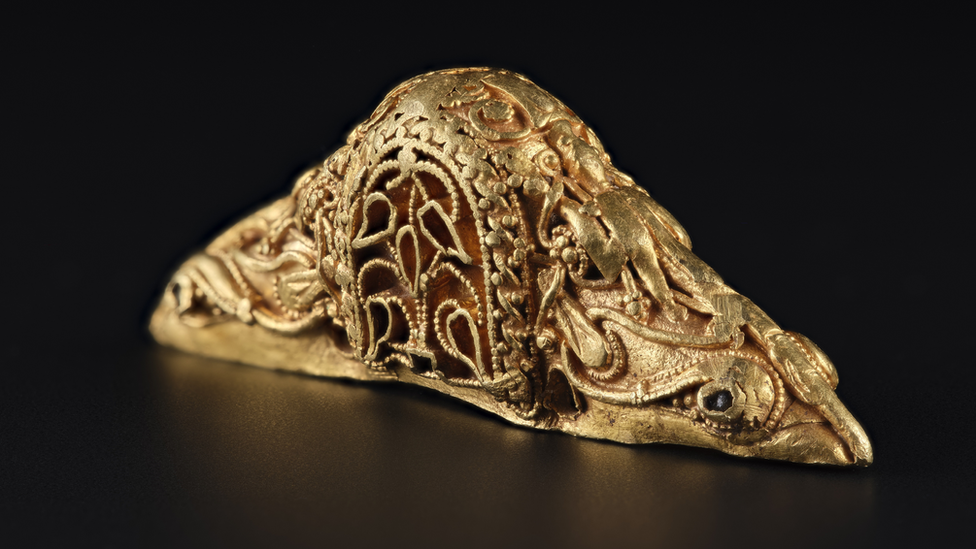The image showcases an elaborate piece of metal artwork, likely from an ancient civilization, displayed on a dark, possibly shiny, surface with a black or very dark brown background. The artifact is gold or brass in color, potentially crafted or painted in that hue. It features a triangular shape with a rounded, arched top and intricate detailing throughout. The center includes an ornate, possibly braided metal archway with delicate designs. A leaf pattern adorns the front center, and towards the right, there are two eye-like structures with black beads within, hinting at the depiction of an animal. The piece has a textured surface and exhibits a flat base, suggesting it could be a statue, decoration, or even a functional object like a bookend.